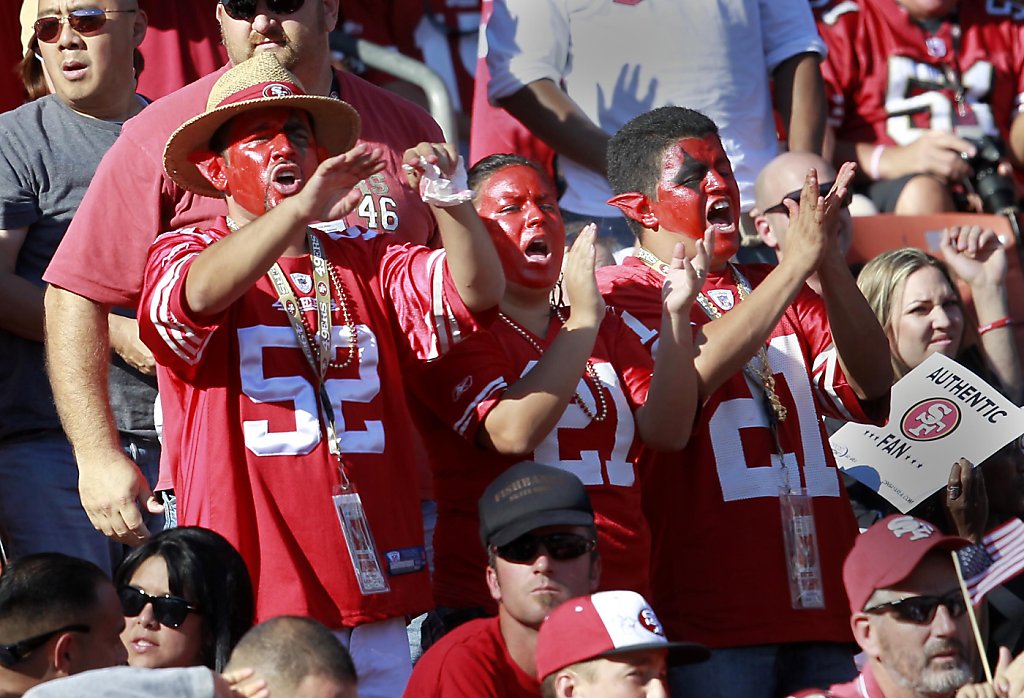In this dynamic photo captured during a sunny San Francisco 49ers football game, the central focus is on three passionate fans prominently positioned in the stands. Their faces vividly painted red like little devils and donned in bright red 49ers jerseys, they stand out due to their infectious enthusiasm. The man on the left sports a number 52 jersey and a straw hat, while the other two—a man and a woman—wear jerseys numbered 21. The woman is positioned in the middle, creating a striking trio. They are all energetically clapping and cheering for their team, starkly contrasting the surrounding fans who appear seated, serious, or otherwise occupied. Just to their right, an "Authentic Fan" sign with the classic red oval San Francisco 49ers logo can be spotted amid the crowd. The scene, bathed in sunlight, suggests a lively game day atmosphere, although it's unclear if the game is happening in San Francisco or elsewhere.